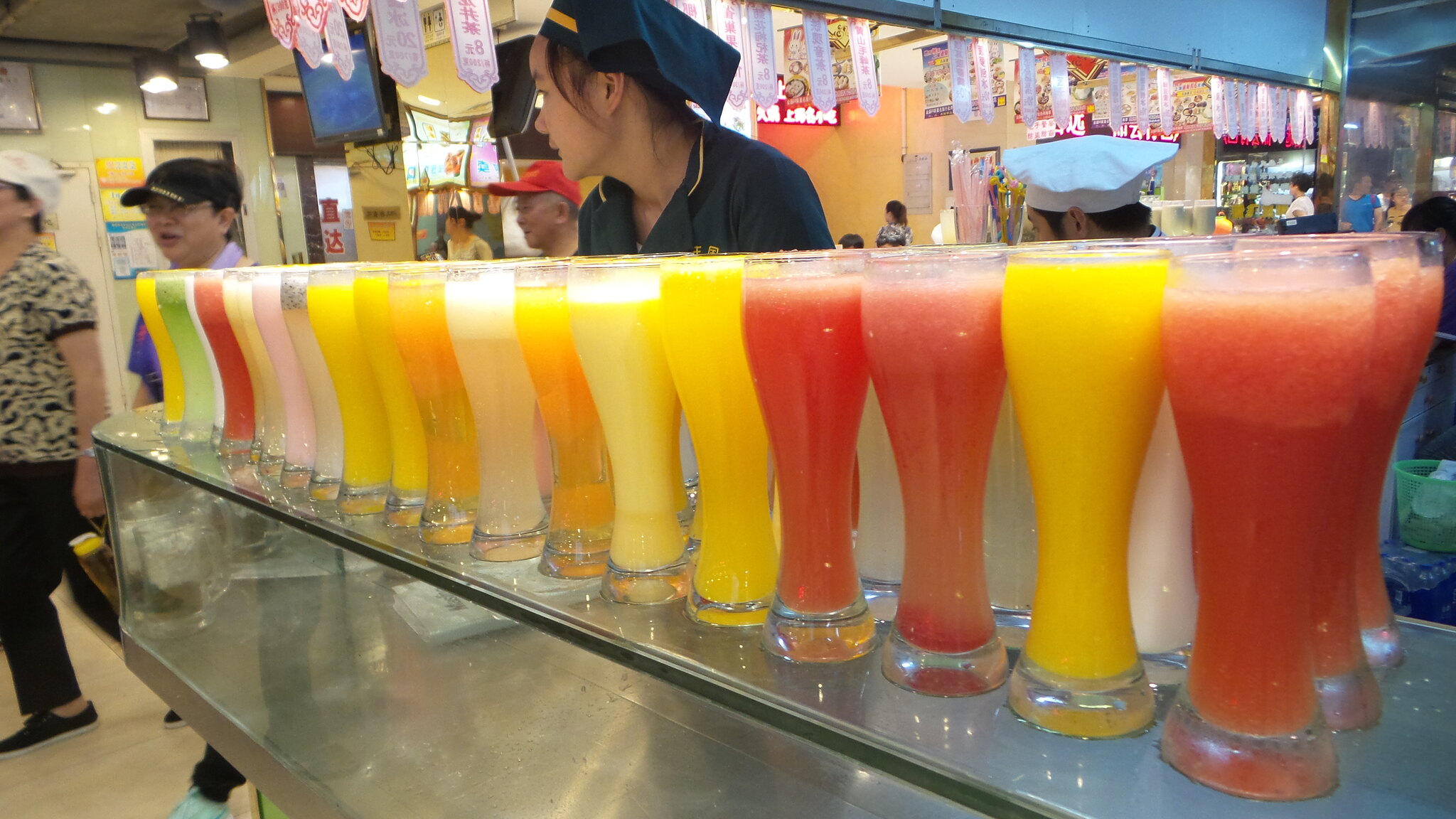The photograph depicts a bustling juice bar, likely located in Asia, as evidenced by the presence of Asian characters and staff primarily of Asian descent. Dominating the foreground, a sleek glass table displays an array of Pilsner-style glasses, each holding a vibrant juice ranging in color from deep reds and blood oranges to yellows, beige, milky whites, and even a lone green on the far left. The glasses, with their narrow bottoms flaring out to wider tops, are neatly arranged in rows of three, extending to form a long, orderly line.

In the background, workers and patrons populate the space. Central to the scene is a woman wearing a blue hat, suggestive of an employee, while other individuals, perhaps customers, mill about. The presence of various uniforms, including a chef's hat and baseball caps adorned with logos, reinforces the bustling, organized atmosphere of the establishment. Hanging from the ceiling, talisman-shaped objects with Chinese characters add a cultural touch, possibly indicating customers' orders or serving a decorative purpose. The overall ambiance suggests a vibrant, well-frequented juice bar or restaurant environment.